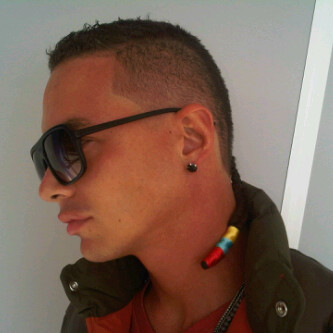This color photograph features a side profile of a young man, possibly Colombian singer J Balvin. He sports a buzz cut on the sides of his head with slightly thicker, brown hair on top. A dark black stud earring decorates his left ear, and he is wearing dark sunglasses. He is dressed in an olive-green, puffy jacket that appears to have a concealed hood, with a red shirt peeking out from underneath. Interestingly, a vibrant, rainbow-colored object—perhaps a wrap for a ponytail—encircles his neck, displaying colors of red, blue, and yellow. The background is a mix of blue and white, suggesting an indoor setting.